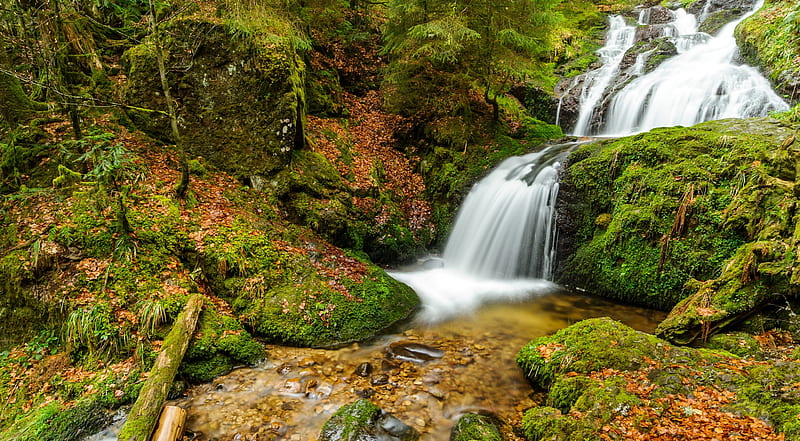This vibrant landscape image captures a serene, woodsy scene dominated by a cascading waterfall. The waterfall originates from the top left of the image, appearing brilliantly white and crystal clear, and flows down two rock tiers covered in deep, dark green moss. The water eventually pools shallowly over a bed of small, shiny rocks before continuing as a stream. The surrounding area is filled with rich, lush greenery, with trees that are either still in bloom or beginning to lose their leaves, hinting at early fall. Moss-covered logs lie scattered around, blending into the predominantly green and brown color palette of the scene. The longer exposure of the photo beautifully captures the ongoing motion of the waterfall, emphasizing the clarity and flow of the water amidst the natural setting.